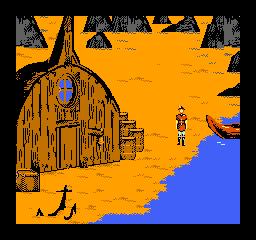In this square image from an old video game with basic graphics, a pirate character stands prominently. The pirate is clad in a detailed red uniform complete with a distinct hat and high black boots. Surrounding the image is a stark black border. To the right of the pirate, a small, canoe-like boat is pulled up onto the shore, barely qualifying as a ship. The bottom right corner of the image features a diagonal expanse of blue water. The rest of the ground is blanketed in warm orange sand, sprinkled with high black rocks. To the left of the pirate stands a wooden shack, its weather-beaten facade adorned with a single circular window above the door and several barrels clustered nearby. The shack, uniformly brown, adds to the scene's rustic feel. Scattered on the sandy ground lies a partially buried ship's anchor, its black iron contrasting sharply with the vibrant sand.